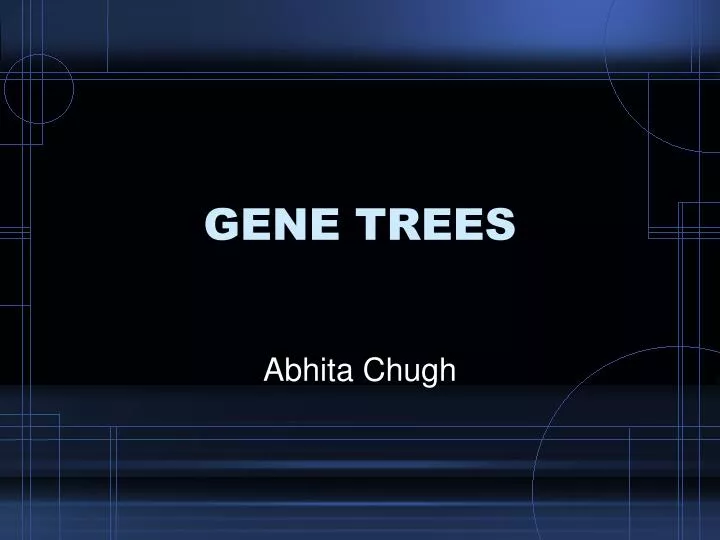The image features a predominantly black center with a subtle blue border. Along this border are intricate, light white lines forming multiple thin, overlapping circles, squares, and rectangles, creating a mesh of geometric shapes and figures. Key shapes include a small circle at the top left, a small circle at the top right, and a larger circle at the bottom right. Additionally, there are various polygons, mainly parallelograms, scattered throughout the image. 

In the middle of the image, in bold, white, all-caps font, the text reads "GENE TREES." Beneath this, and also centered, is the name "ABHITA CHUGH" in white font. The geometric figures and lines frame the central text from the top, bottom, and sides, adding a detailed structure to the otherwise simplistic design. The image appears to be a computer display page, possibly serving as a title or start screen for a presentation, with a focus on the visual appeal of genetically produced trees.